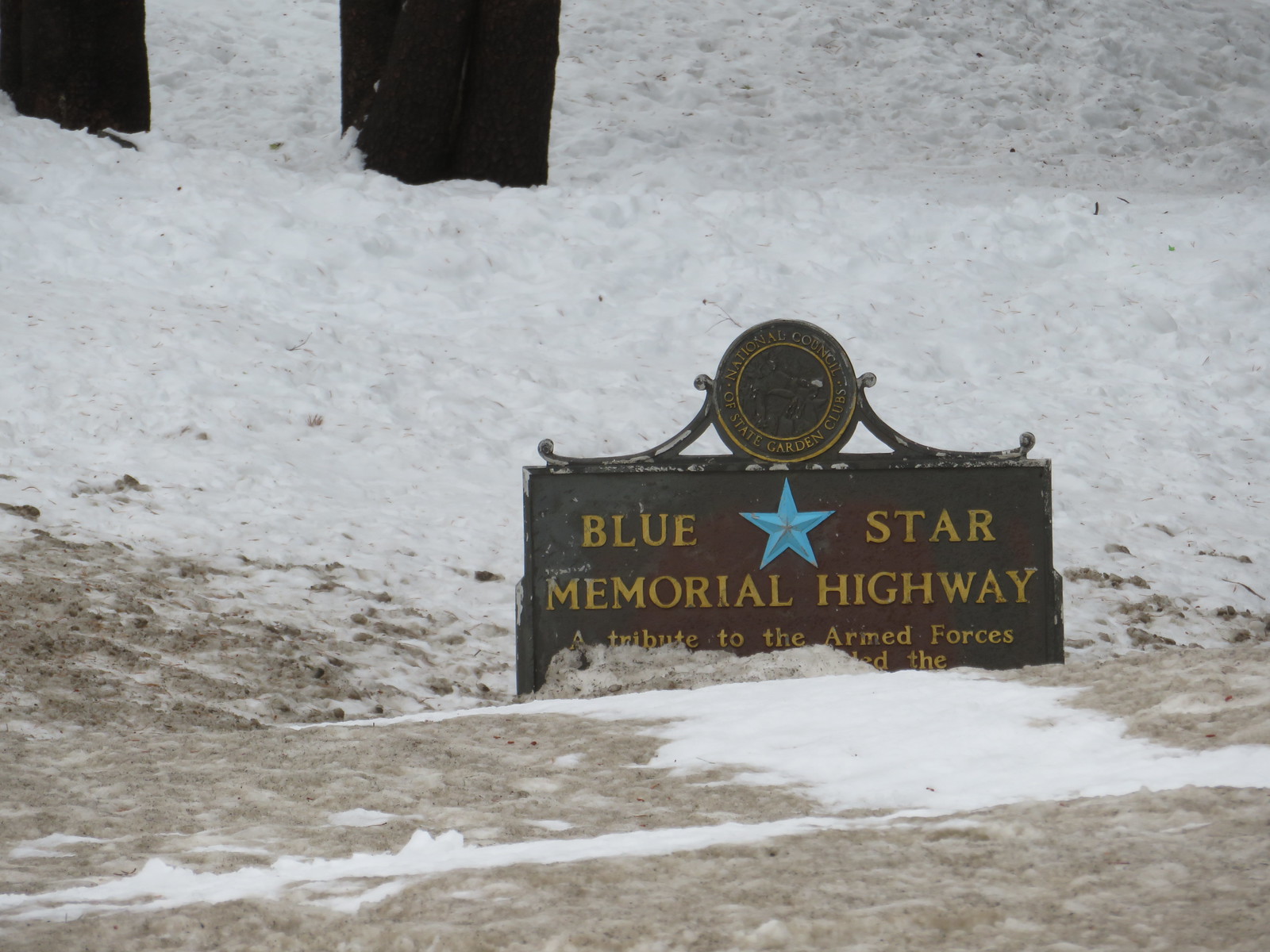In this photograph, a heavily snow-blanketed scene sets the backdrop for a prominent signpost. The sign, an olive or dark-colored plaque with gold lettering, reads "Blue Star Memorial Highway," honoring the armed forces. A distinct blue star is positioned between the words "Blue" and "Star," while the sign's top features a circular seal inscribed with "National Garden Clubs." The sign appears partially obscured, either broken or buried in snow, with just the initial tribute words visible. Below the sign, snow covers a stone staircase that leads downwards, bordered by tree trunks that peek out from the wintry field. The landscape, dominated by a pristine snowy expanse, transitions to a dirtier snow near the ground, completing this serene yet somewhat desolate winter scene.